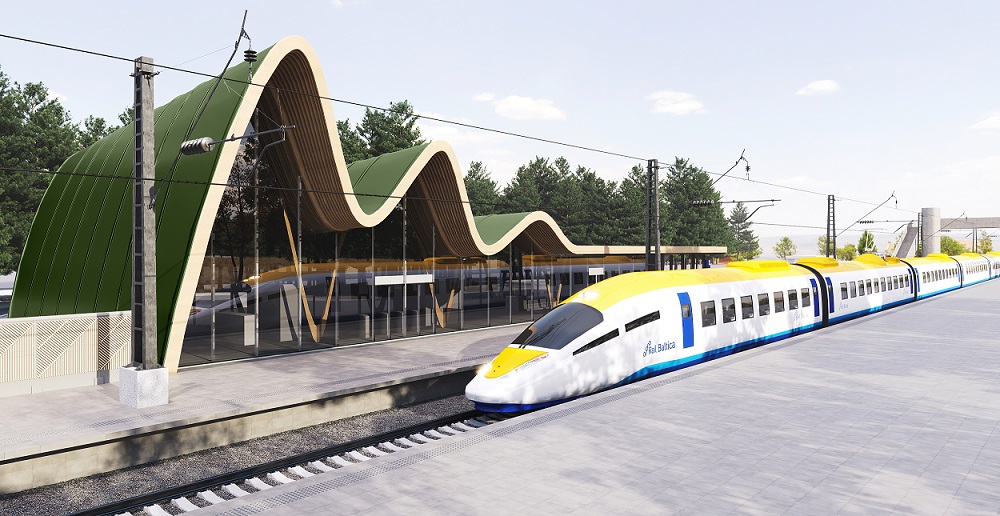The photograph captures a bustling train station with a prominent view of the train, tracks, and platforms. Dominating the foreground, the train is a sleek, heavily curved design, with a distinctive yellow roof, white sides, and blue lower sections and doors. It runs on neatly laid black rails flanked by white boards and gravel.

On the bottom right corner of the image, there lies a flat, gray-tiled pedestrian area, mirrored by a smaller, similarly tiled platform on the opposite side. These platforms are bisected by the train tracks running down the center of the image.

In the background, to the left, there is a cluster of tall, lush green trees that extend more than halfway through the image, gradually giving way to smaller trees and bushes. Looming over the platforms on the left side is an abstract, curvy, green-roofed building with glass walls, through which various seating areas are visible. This glass building appears reflective, with metal beams and wires adding to its modern aesthetic.

A cylindrical structure with a catwalk and stairs is also visible in the far back, providing depth and context to the station's complex layout. Above it all, the sky stretches across the entire top part of the image, fading to white as it reaches the horizon.